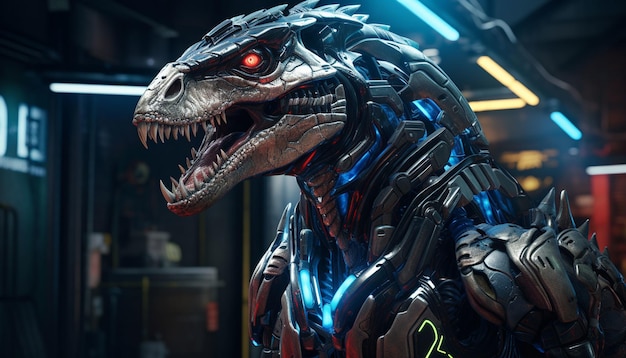The image showcases a highly detailed, metallic robotic dragon, gleaming with a silver and gray metallic surface. Its large, menacing mouth is agape, revealing sharp teeth in both the upper and lower jaws, while a detached jaw structure emphasizes its fearsome appearance. The dragon's single, glowing red eye contrasts starkly against its shiny exterior. Along the top of its head and extending down the neck are spine-like structures resembling horns. Interspersed within the metallic framework are neon blue accents, with blue light emanating from the chest and neck joints, hinting at an internal illumination. The creature is oriented towards the left side of the image, emphasizing its articulated neck connections. The background appears to be a blurred scene reminiscent of a warehouse, softened by a bokeh effect with diffused blue, yellow, and red lights scattered throughout. A particular red and white blurred object is noticeable on the right side of the frame, adding to the complex, industrial ambiance.